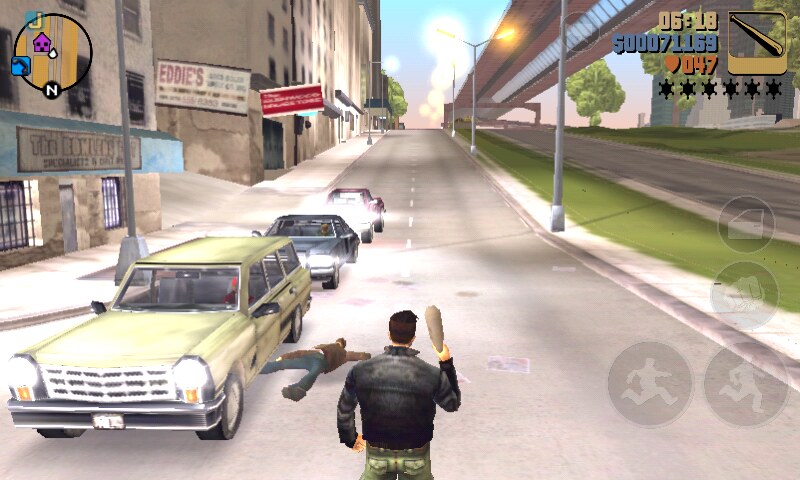The screenshot depicts a scene from a video game with simplistic rendering. In the center, a muscular man with brown hair is holding a club in his right hand. He is dressed in a black leather jacket and matching pants. On the left side of the road, three cars are parked in a row: a yellowish box car, a gray car behind it, and a red truck. A man is partially lying under the yellowish box car. The background features tall, gray buildings housing various shops and businesses. On the right side of the road, there is a green median with sidewalks flanking it, along with several streetlights. A red overpass is visible overhead. In the top right corner of the image, a bat logo is prominently displayed.